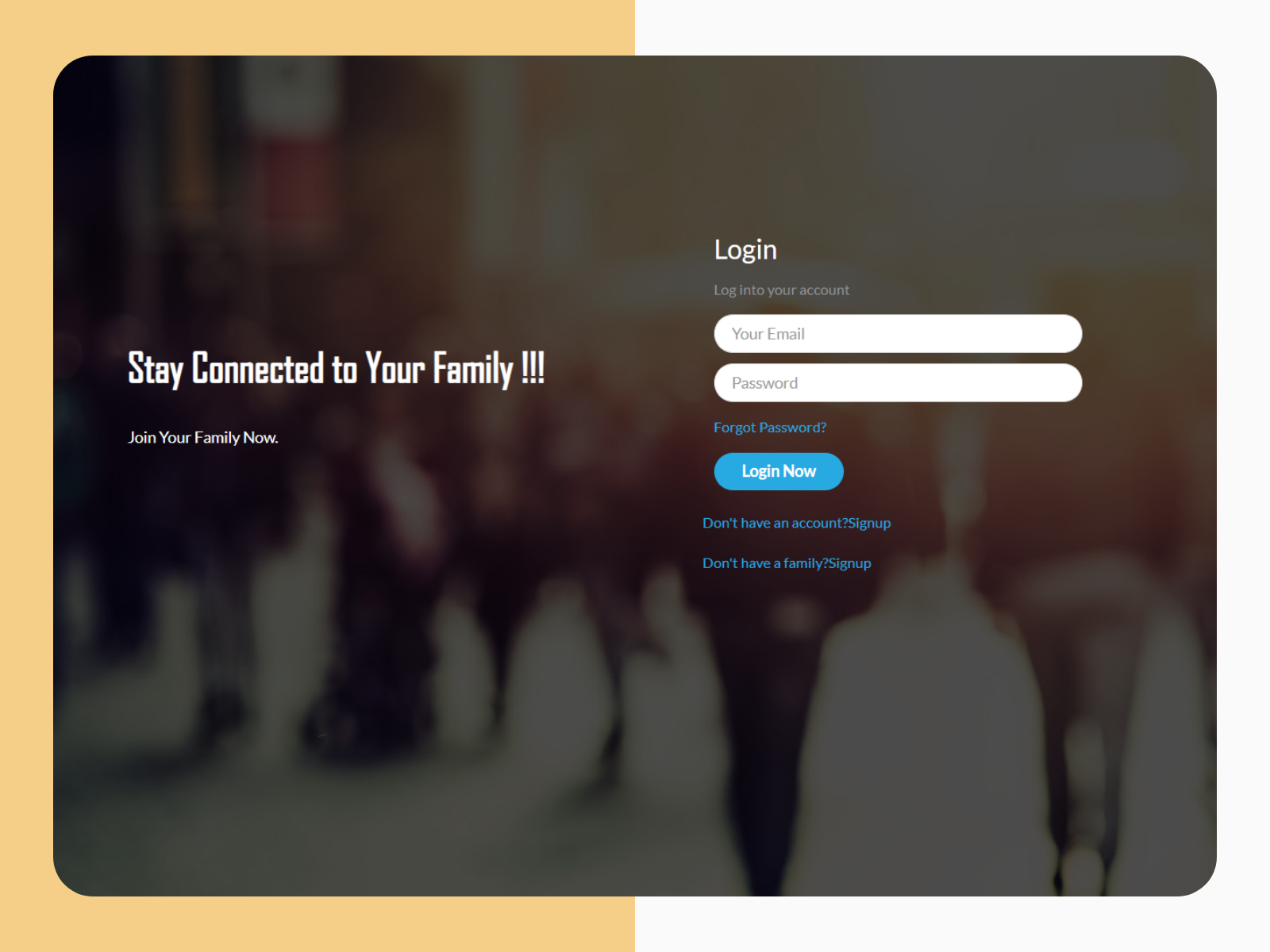The image is a detailed screenshot of a login page, presented in a landscape orientation. The background of the image is divided vertically into two sections. The left side features a light orange hue, while the right side transitions into a light gray, almost white shade.

Within this image is a prominent, large rectangle with rounded edges, serving as the main focal point. The rectangle's background displays a blurred, filtered photograph of people walking on a city street. Due to the blurriness and the muted, sepia-toned colors at the top transitioning to darker grayish hues at the bottom, only general outlines of the individuals are discernible. Among these figures, one person appears to be pushing a stroller, and two women seem to be walking away from the viewer on the right side of the image.

Overlaying this background are various pieces of text and interactive elements. On the left side of the rectangle, white text reads, "Stay connected to your family!!!" followed by the invitation, "Join your family now." On the right side, the text prompts the user with, "Log in to your account." Below this are two input fields: one for the user's email and the other for the password. Just beneath the password field, there is a "Forgot password?" link in blue text. At the bottom of the login section is a blue button with white text that reads, "Log in now."